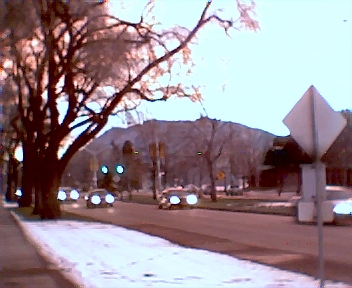In this somewhat blurry photograph with a purplish pink tint, we see a suburban street scene taken during wintertime at dusk. The street is lined with bare trees, snow dusting the grass and filling the ditch area along the road. A sidewalk runs parallel to the street, bordered by patches of snow. In the background, there is a view of a small mountain or large hill under a hazy sky. Cars are driving toward the camera, their headlights cutting through the dim light despite the moderate daylight still present. A green traffic light is visible in the distance. On the right side of the image, the backside of a street sign is visible, showing only its metal parts, while another sign can be faintly seen further away. To the left, a larger tree stands out with a single branch sticking out at a 45-degree angle. The overall impression is of a quiet winter scene in a suburban area, with elements of nature and infrastructure intermingling under a slightly surreal, tinted sky.